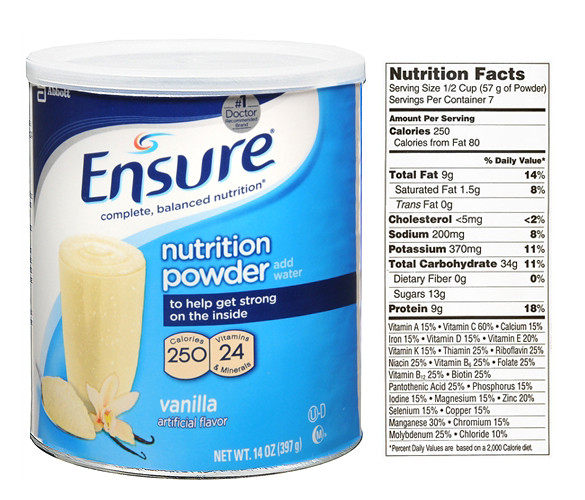The image displays a can of Ensure Nutrition Powder against a white background that appears to be edited for clarity. The can features a design with darker blue at the top, a white strip in the middle, and the majority of the can in light blue. Prominently displayed on the can are the words "Ensure Complete Balanced Nutrition" alongside the slogan "Add water to help get strong on the inside." The can contains 14 ounces (397 grams) of vanilla artificially-flavored powder. Each serving, approximately half a cup, offers 250 calories and includes 24 vitamins and minerals. Nutrition facts summarized on the side indicate each serving contains 9 grams of total fat, 200 milligrams of sodium, 370 milligrams of potassium, 34 grams of carbohydrates, 13 grams of sugar, and 9 grams of protein. The image also highlights a white drink with a vanilla flower beside the can, enhancing the vanilla theme. The overall presentation is designed to emphasize the product's nutritional benefits, appealing to those seeking a balanced dietary supplement.